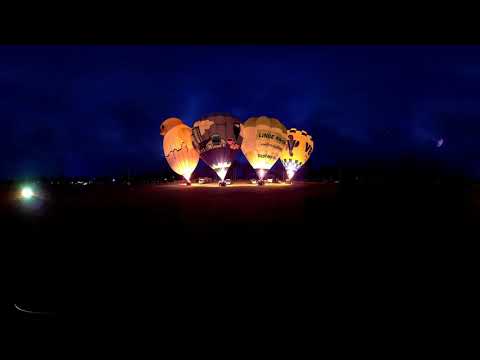The image captures a mesmerizing nighttime scene featuring four hot air balloons, all aglow from the flames that light them up from within. The sky is a deep navy blue, adding to the dramatic effect created by the fiery illumination of the balloons. Positioned approximately a football field's distance away, the balloons are lined up on the ground with their baskets resting below them. 

Three of these balloons have a predominantly yellow hue, while the second one from the left stands out with its purple color. The leftmost balloon has an orange-like tint and is topped with a whimsical rubber ducky head. Despite the low resolution, vague details of sponsorship logos or cartoon characters are visible on the balloons. The two rightmost balloons display business logos. Additionally, there's a small bluish light toward the left side, seemingly unrelated to the balloons, possibly from distant buildings.

Nestled in the dark surroundings, these glowing giants create a stunning visual highlight against the black foreground and slightly clouded night sky, reflecting the magical essence of a hot air balloon show. There's no crowd visible in the image, suggesting a quiet moment before or after the main event, adding to the serene yet striking ambiance of this midnight spectacle.